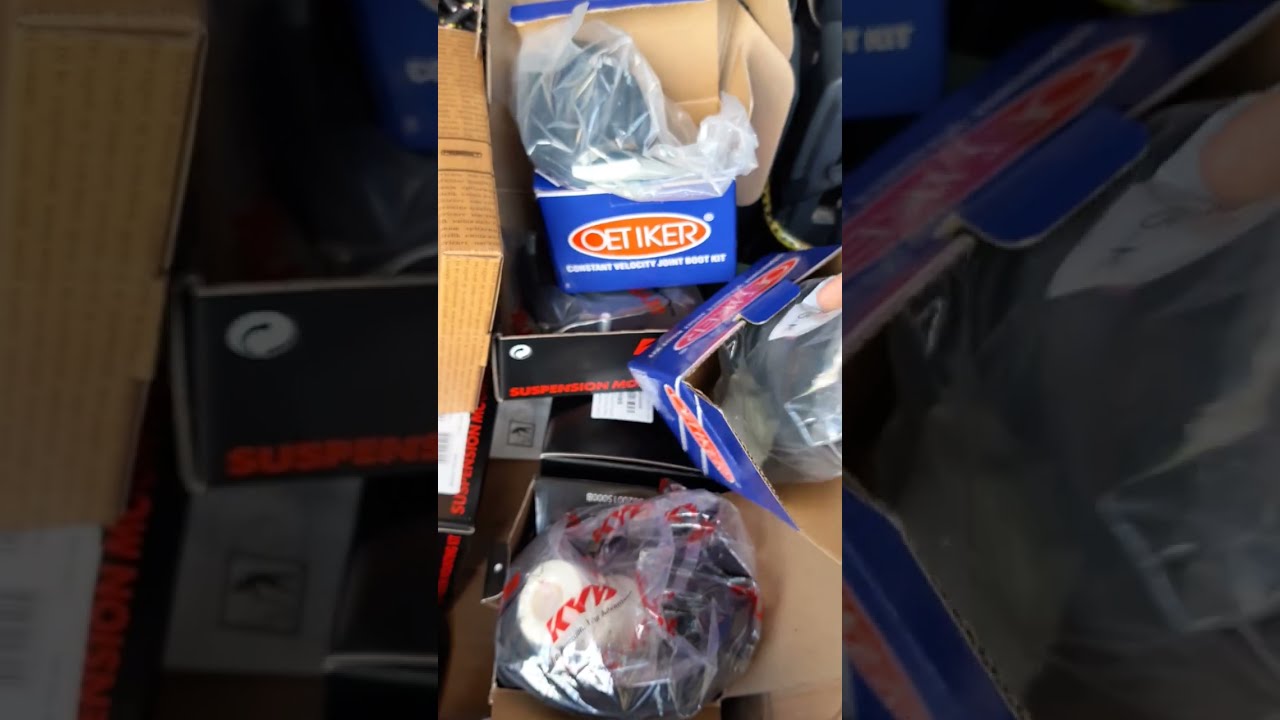The image captures a slightly out-of-focus, small cell phone photograph depicting a collection of various automotive product boxes, many of which are open. Central to the image is a blue rectangular box prominently displaying the brand name "OETIKER" in white lettering inside an orange oval logo. Positioned on top of a black rectangular box labeled with the word "suspension" in red, the blue OETIKER box, likely containing brake pads or accessories, sits among an assortment of other packages. Beneath these, there is a brownish-beige background which might resemble a car seat. Scattered around are additional boxes, some revealing contents still encased in plastic bags, one of which is partially labeled "K-Y." The image overall suggests that the boxes contain various car accessories, including a "Velocity Joint Boot Kit," looking somewhat jumbled as if they have been hastily collected or unpacked. The photo also features blocks on the left and right showing enlarged sections of the main photo, adding to the somewhat cluttered and unclear presentation.